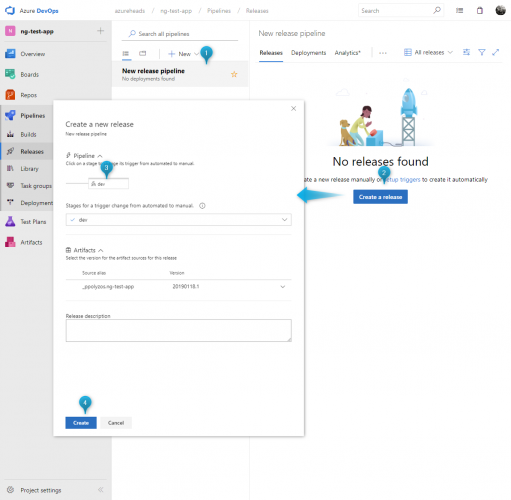The image is a slightly taller than wide screenshot of a web page, likely from a platform related to Azure DevOps. In the upper left corner, there's a small blue icon resembling a TV or square box, followed by the word "Azure" in black text and "DevOps" in blue text. The top menu bar has four items in gray text, with the last one seemingly labeled "Releases," although they are quite blurry.

On the far right of the top menu is a search box with a gray magnifying glass icon, two additional icons, and a profile picture at the very end.

Along the left side of the screenshot, there is a vertical menu. The first item is labeled "NG Test App" and features a purple icon with a white "N" in it. This is followed by an "Overview" tab, then "Boards," and possibly "Properties" (though the label is unclear). Subsequent menu items include "Builds," "Releases," "Library," "Task Groups," "Deployments," "Test Plans," and "Artifacts." Each menu item is accompanied by its respective icon.